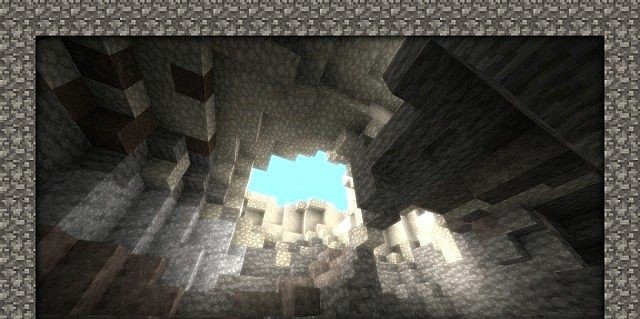This Minecraft image captures the interior of a cave, showcasing its blocky, pixelated charm. From the vantage point inside the cavern, you can see a circular hole in the cave’s ceiling, through which a vibrant, turquoise sky is visible, offering a stark contrast to the dimly lit cave below. The cave itself is constructed from various small, uniform cubes, each one featuring distinct colors and textures that combine to create a more complex, natural appearance. Surrounding the central image is a low-resolution frame, echoing the basic textures of the cave with its gray coloration interspersed with darker and lighter streaks. This framing adds to the overall aesthetic, giving it a polished yet rugged look. The detailed texturing and strategic mix of cubes enhance the realism within the otherwise uniformly structured world of Minecraft.